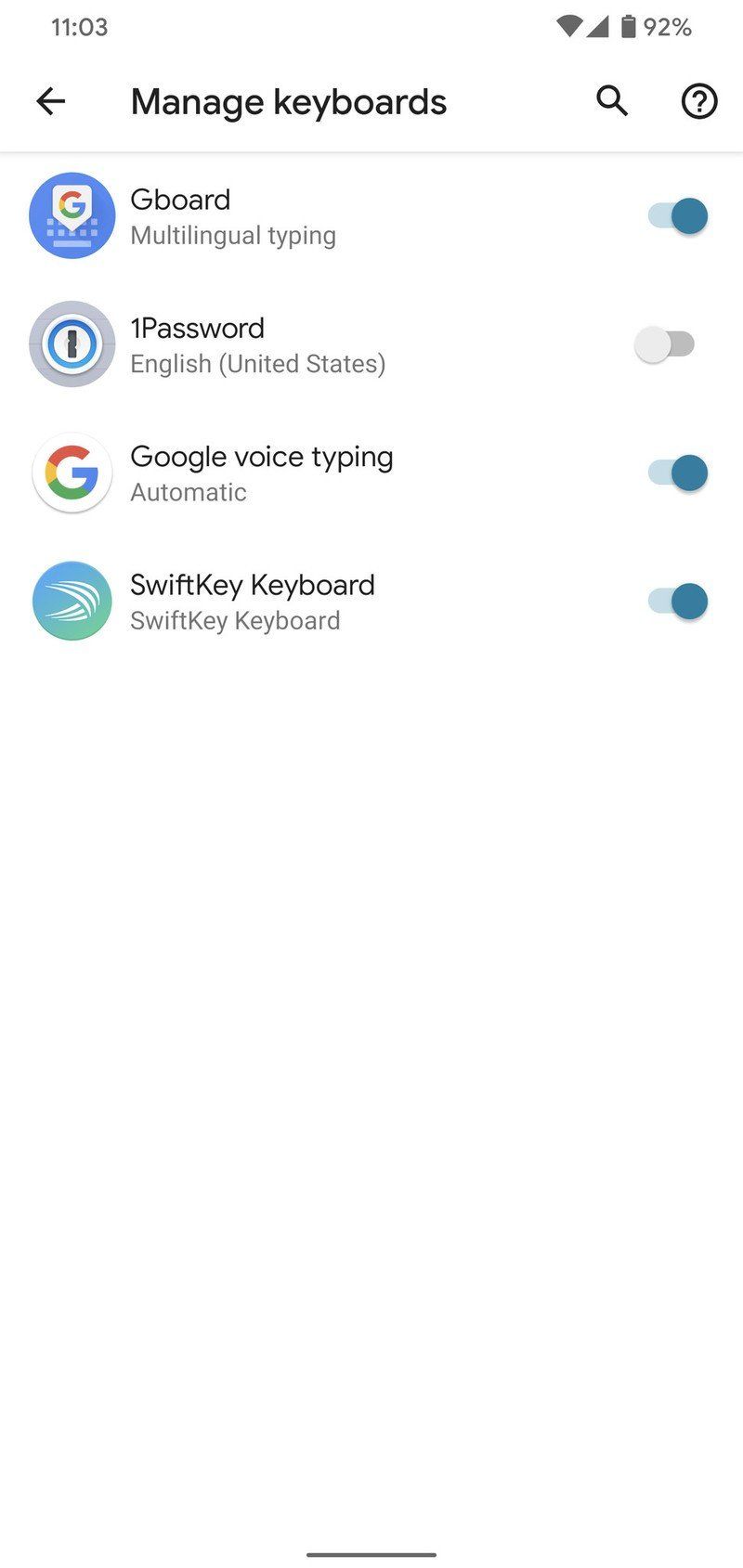A mobile screenshot captures the settings menu of a managed keyboard on a white background. The top portion of the screenshot displays standard mobile status icons with the time at 11:03 on the upper left. On the upper right, the status icons include a signal strength indicator resembling a pie slice, a cell strength right triangle, and a vertically oriented battery icon showing 92% charge.

Immediately below the status bar, an arrow points left, leading to the headline "Manage keyboards," which is accompanied by a search magnifying glass and a help icon (question mark inside a circle). The menu lists four distinct keyboard settings.

1. **Gboard:**
   - **Icon:** Blue circle with a keyboard symbol light blue in color, featuring the Google "G" inside a white quotation box.
   - **Label:** Gboard
   - **Subtext:** Multilingual typing
   - **Status:** Enabled (teal-blue slider with the circle to the right)

2. **1Password:**
   - **Icon:** Blue-outlined white circle with a vertical line (like an "I" or "1"), resembling a bullseye.
   - **Label:** 1Password
   - **Subtext:** Not provided
   - **Status:** Disabled (gray slider with the circle to the left)

3. **Google voice typing:**
   - **Icon:** Google "G"
   - **Label:** Google voice typing
   - **Subtext:** Automatic
   - **Status:** Enabled (teal-blue slider with the circle to the right)

4. **SwiftKey Keyboard:**
   - **Icon:** Circle with a gradient background (sky blue on the upper left and green on the bottom right) featuring white arched stripes, resembling a folded handkerchief.
   - **Label:** SwiftKey Keyboard
   - **Subtext:** SwiftKey Keyboard
   - **Status:** Enabled (teal-blue slider with the circle to the right)